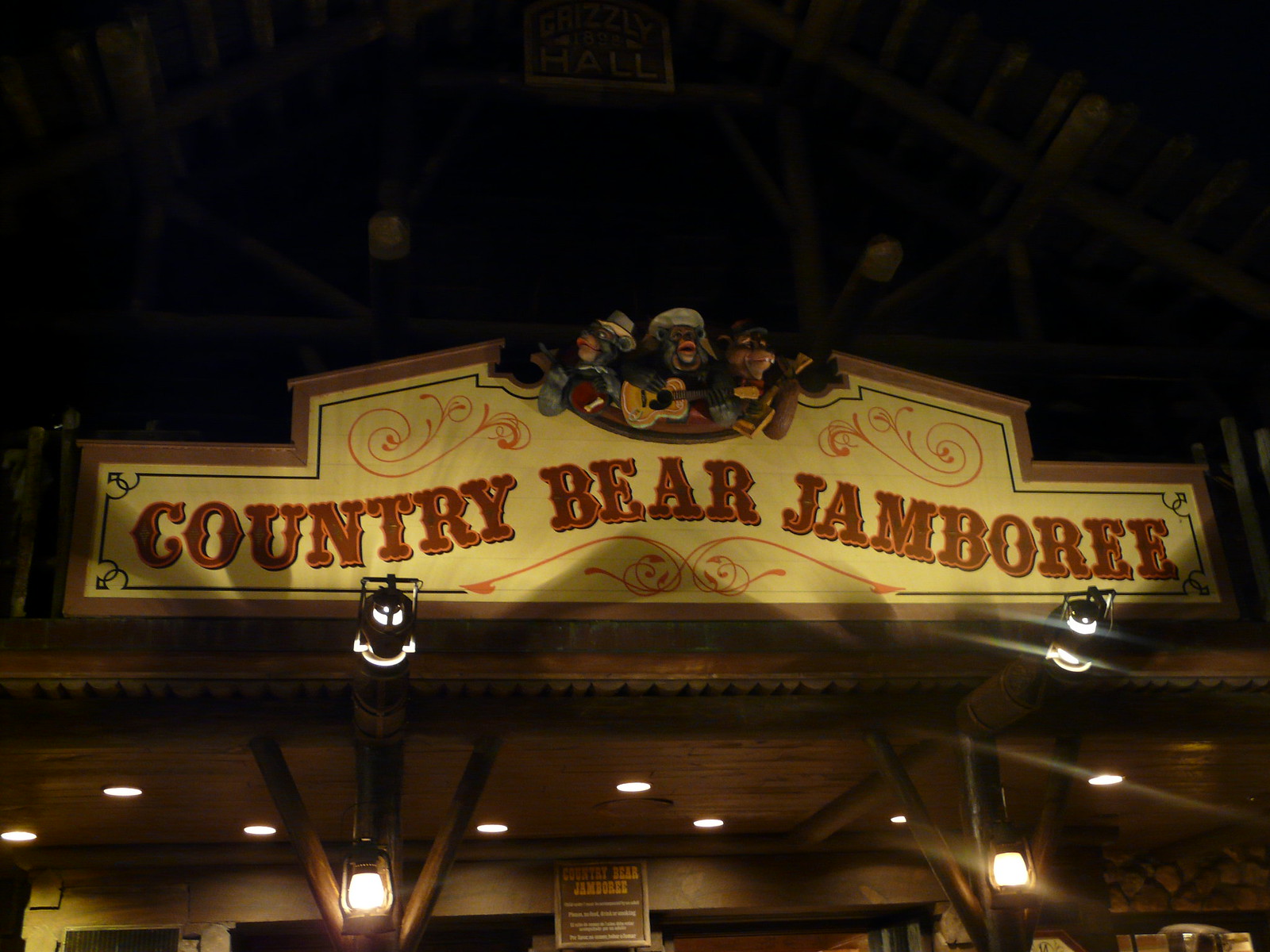This nighttime image captures the front of a business with an old Western wooden façade. The photo is taken from a low angle, pointing upwards, showcasing the building's porch ceiling with recessed lighting and two wooden posts supporting rafters with lit lanterns hanging from them. At the bottom of the image, the entrance is partially visible, illuminated by stage lights.

The focal point is the large marquee sign on the roof, which reads "Country Bear Jamboree" in capital brown letters with an orange outline, styled in an old Western font. Decorative, swirling lines embellish the sign. Atop the banner, three animatronic bears are depicted playing instruments. The central bear faces forward, while the bear on the right looks right and has buck teeth, and the one on the left looks left. Two bears appear to be playing guitars, while the one on the far right plays a banjo. Overall, the scene has a charming, nostalgic atmosphere, hinting at an interesting attraction worth exploring further.